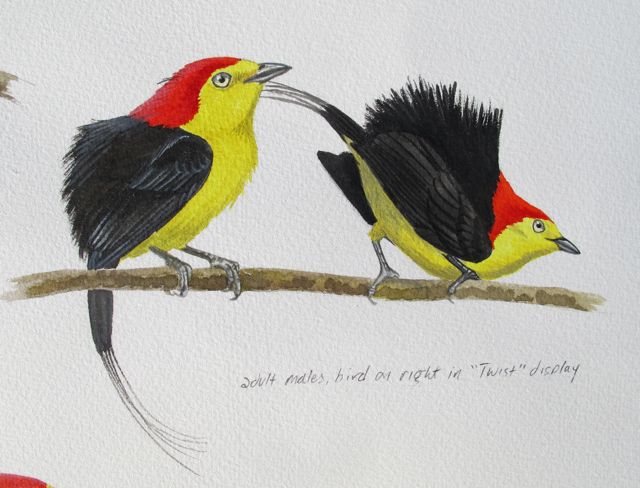The image features a detailed drawing of two vibrant wire-tailed manakin birds perched on a horizontal, leafless brown branch against a clean white background. Beneath the branch, text scrolls that read: "Soulmates," and "Bird on right in twist display." The first bird on the left, with bright red plumage on the top of his head, has yellow coloring on his face and breast, black feathers covering his back and the rest of his body, and gray feet gripping the branch. This bird appears relaxed, looking upwards with a gray beak and eyes that alternate between black and yellow. In contrast, the second bird on the right, similar in coloration, has his tail lifted and appears to be dipping downward, possibly focused on an unseen object. The artwork employs a limited color palette of predominantly yellow, red, and black, with touches of gray, brown, and white, resulting in a striking visual composition.